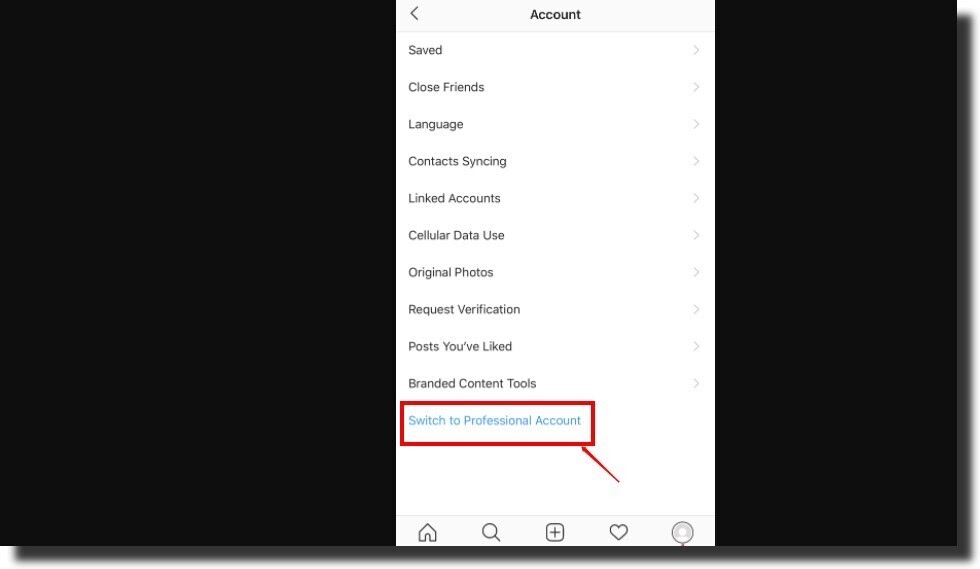This image appears to be a screenshot captured from a phone, nestled within a larger image. The outer frame of the image is completely black, resembling a long rectangle. A discernible shadow is cast along the right-hand side, extending downward and continuing along the bottom border, nearly reaching the left bottom corner.

Centrally positioned in the black background is the phone screenshot. This screenshot features a light gray box in the center, labeled "Account," accompanied by an arrow pointing to the right. Below this box, the background turns white, showcasing a list of various options in rows. Each row commences with an arrow pointing to the right on the left side. The following rows are listed: "Saved," "Close Friends," "Language," "Contacts Syncing," "Linked Accounts," "Cellular Data Use," "Original Photos," "Request Verification," "Posts You’ve Liked," and "Branded Content Tools."

Highlighting the list at the bottom in red is the text "Switch to Professional Account," making it stand out prominently against the white background.